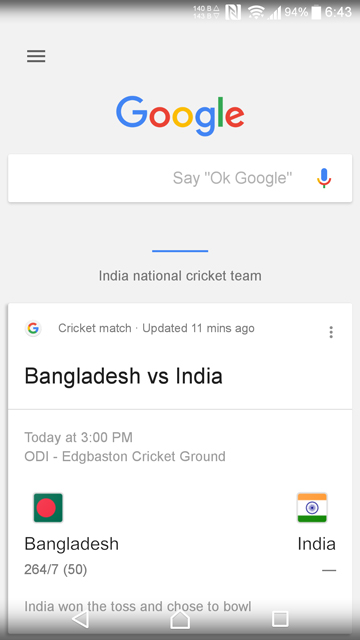The image depicts a smartphone screen displaying a Google search results page. At the top center of the screen, the colorful Google logo is prominently featured, with the letters "G" in blue, "O" in red, "O" in yellow, "G" in blue, "L" in green, and "E" in red. In the top-right corner of the screen, the status bar shows the battery level, the current time, and the Wi-Fi connectivity icon. On the top left, there are three horizontal gray lines representing a menu icon.

Below the Google logo, there is a white search bar with the prompt text "Say 'OK Google'" in gray, accompanied by a small microphone icon to the right of the text. Beneath the search bar, a blue divider line separates the search field from the main content.

The main content headline reads, "India National Cricket Team," followed by a cricket match update posted 11 minutes ago. The update details the ongoing match between Bangladesh and India. The text "Bangladesh vs. India" appears in large black font.

Further down, there is a horizontal line, followed by today's match schedule at 3 p.m. The match is identified as an ODI (One Day International) taking place at Edgbaston Cricket Ground. The team flags are displayed: Bangladesh on the left with a green field and a red circle, and India on the right featuring three horizontal stripes—orange on top, white with a blue Ashoka Chakra in the middle, and green on the bottom. The score update below the flags indicates "264/7 (50 overs)," and it notes that India won the toss and chose to bowl.